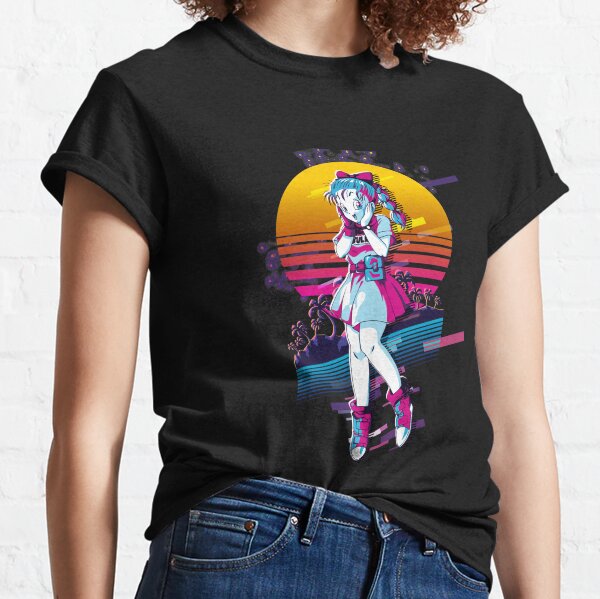This photograph showcases the torso and upper lower body of a light-skinned woman, identified by her curly brown hair, fair neck, and white arms. She is standing against a white brick wall, wearing a black t-shirt with folded short sleeves and blue, tight-fitting jeans that reveal the belt loops, brass button, and front watch pocket. The t-shirt prominently features a circular logo in the center, depicting a cartoonish anime-style girl with blue hair adorned with a pink bow, and a white face with an open-mouthed expression. She is dressed in a purple and blue outfit, with white legs and purple and blue shoes extending above the ankle. Encircling the character is a yellow sun with bright pink and orange stripes radiating through, behind which are silhouettes of palm trees and rocks. A portion of the t-shirt is tucked into the jeans, providing a casual yet detailed look.